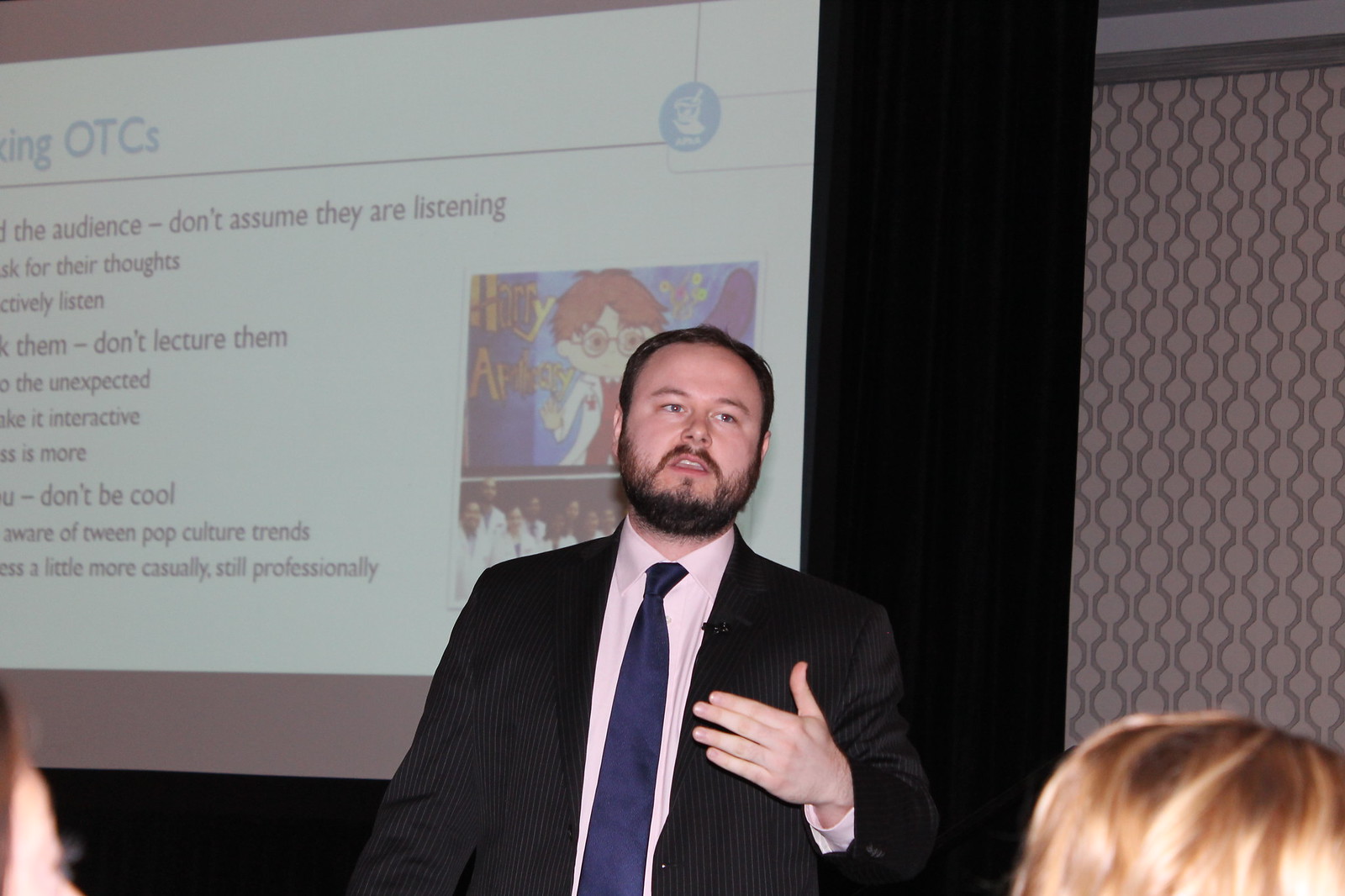The image captures a Caucasian man in a dark pinstriped suit, a tan shirt, and a navy blue tie, standing at a podium or stage, seemingly in the middle of giving a presentation or seminar. He has short brown hair, a mustache, and a beard, and is gesturing with his left hand placed near his chest. He is positioned in front of a large screen, which displays a partially visible slide. The slide features a caricature and text discussing audience engagement strategies, urging not to assume audience attention, not to lecture, making the session interactive, understanding tween pop culture trends, and avoiding attempts to be overly "cool." The words “OTC” headline the slide. The corners of the image show the tops of attendees' heads, emphasizing the interactive nature of the event.